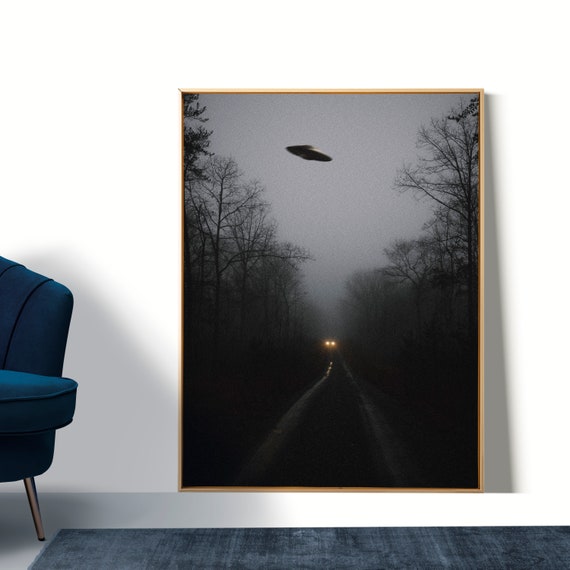The image depicts a framed, black and white photograph that stands vertically against an off-white wall. The photograph, encased in a narrow, gold frame, showcases an eerie scene of a foggy road flanked by spooky, leafless trees. In the distant center of the scene, two amber headlights pierce through the gloom, belonging to a vehicle approaching on what appears to be a dirt or dimly lit road. Hovering above the car is a classic flying saucer, adding a mysterious and unnerving element to the composition. The room's setting includes a blue carpet at the bottom, and to the left, a partial view of a navy blue chair with slender silver legs suggestive of mid-20th century design. The overall atmosphere blends a sense of the paranormal with a nostalgic aesthetic.